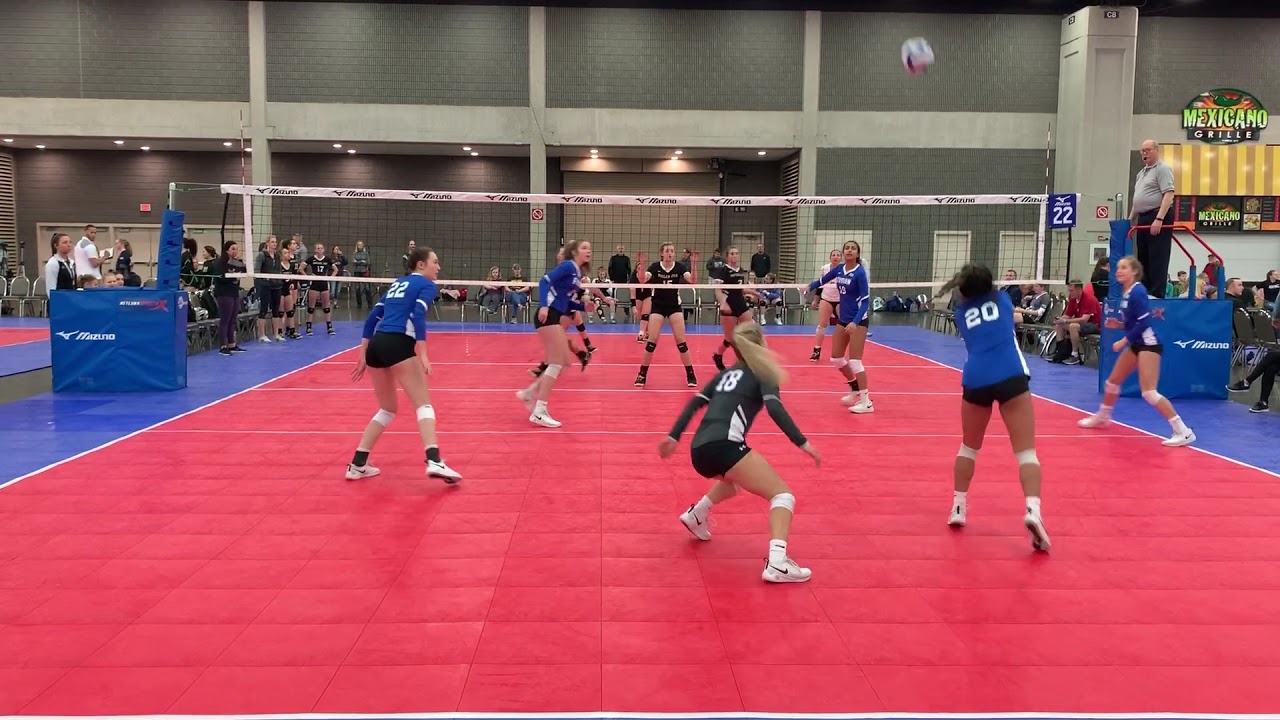The image depicts an intense indoor volleyball match set in a spacious arena. Dominating the center is the volleyball court, flanked by two blue pillars that support a white-trimmed black net. The team closest to the front is clad in blue jerseys, black shorts, and white tennis shoes, while the team on the far end dons all-black jerseys and shorts. A volleyball is suspended mid-air to the upper right, indicating dynamic play. The floor of the court is red with blue boundaries, and the referee stands attentively on the right. Spectators encircle the court, adding to the vibrant atmosphere. In the upper right corner, there's a Mexicano Grill sign, hinting at a nearby restaurant area. The far back wall is dark grey, featuring concrete support pillars that provide an industrial feel. The building's walls are adorned in varying shades of grey, adding contrast and depth to the expansive setting.